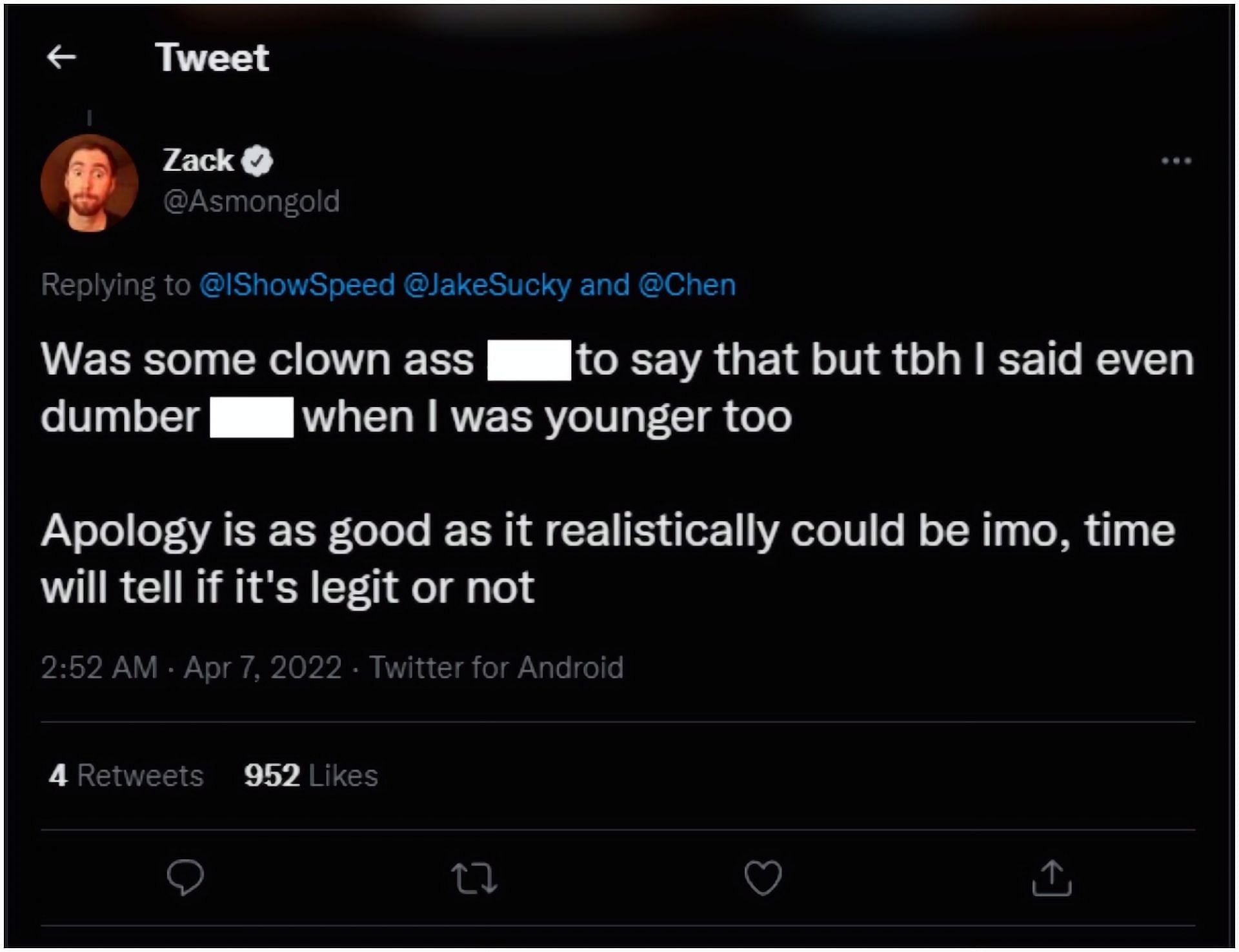**Detailed Caption**:

This tweet, posted by a user named Zach under the handle @Asmongold, prominently features a picture of Zach himself. In the image, Zach sports a beard and mustache, and his eyes appear noticeably wide. He is replying to @ishowspeed, @JakeSucky, and @Chen, whose usernames are highlighted in blue, while the rest of the text is displayed in white.

In his tweet, Zach writes: "Was some clown ass ####, but to be honest, I said even dumber #### when I was younger too. Apology is as good as it realistically could be in my opinion, time will tell if it's legit or not." The censored words are obscured by white blocks.

The tweet was posted at 2:52 a.m. on April 7th, 2022, via Twitter for Android. Since it was posted, the tweet has garnered 4 retweets and 952 likes. Below the tweet, the standard Twitter interaction icons are displayed: a speech bubble for replying, a heart for liking, and a circular arrow for retweeting. Additionally, there is an icon for sharing, which is depicted with two arrows pointing in different directions. At the top of the interface, three horizontal lines indicate a menu option.